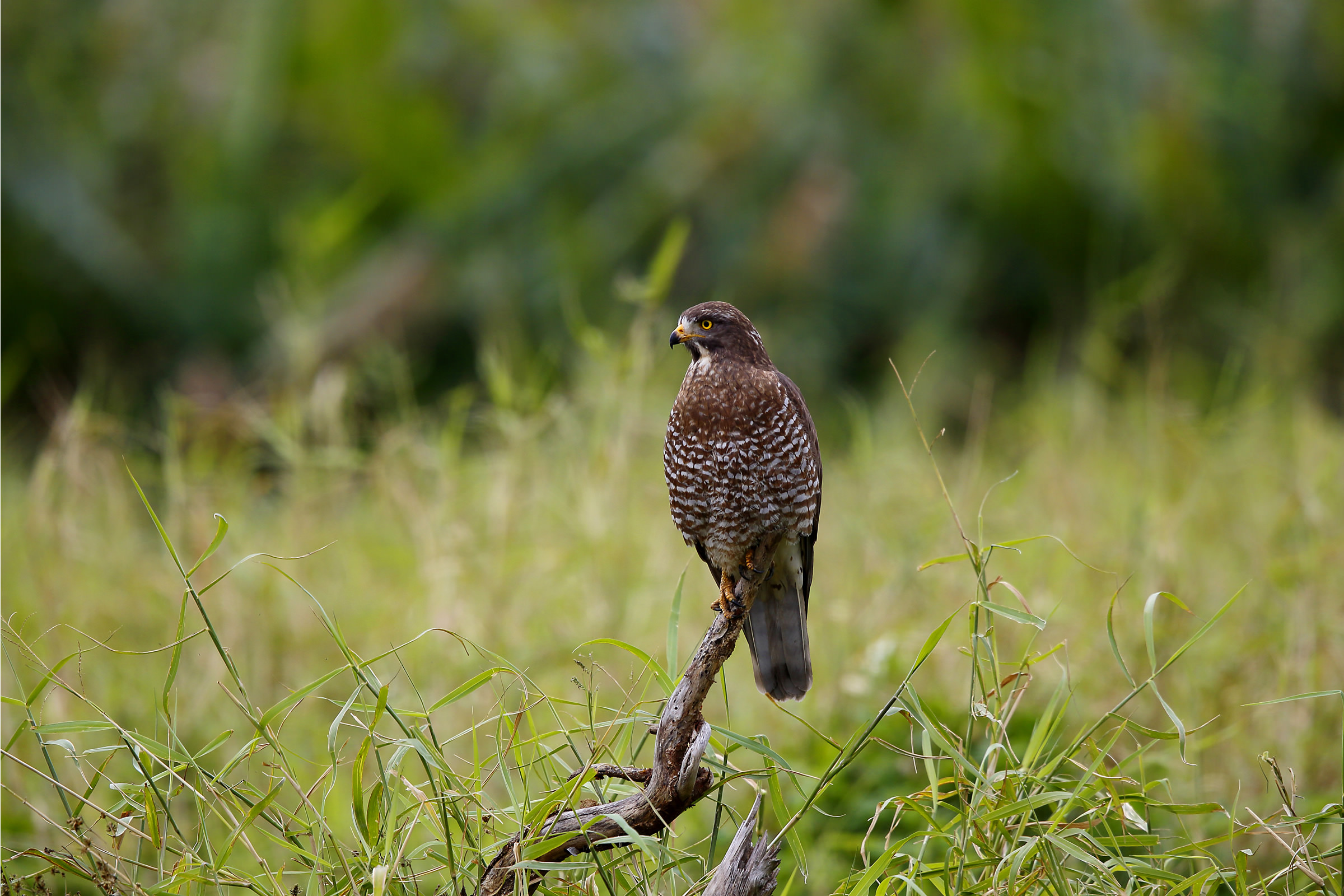This professional wildlife photograph captures a striking bird of prey, likely a Cooper's Hawk or a Peregrine Falcon, perched on a dead wooden limb amidst tall grasses. The hawk, centered in the photograph, features a striking appearance with a red breast, white checking along its belly, and a distinctive black-tipped white underside of the tail. Its plumage is a mix of brown and white, and it has an orange-yellow beak with a black tip. The hawk’s eyes are golden-orange with a black pupil, and its orange feet grip the branch firmly as it gazes into the distance. The background is beautifully blurred, drawing focus to the hawk and the surrounding short greenery, with various shades of green and touches of brown creating a serene outdoor setting.